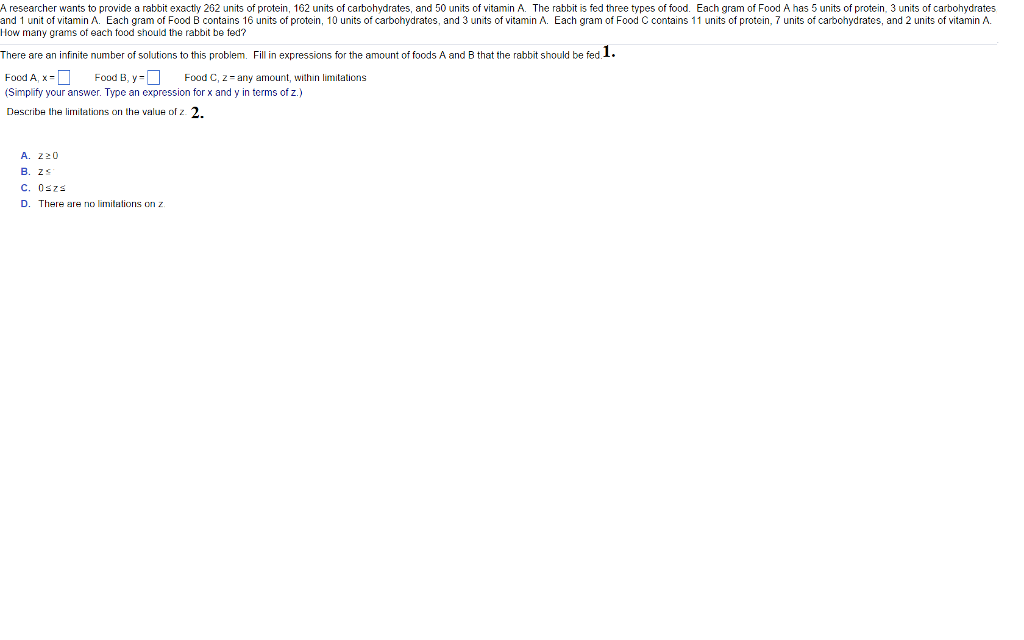**Screenshot Description:**

The image is a screenshot of a math problem presented on a white background, divided into two sections by a horizontal line border.

**Top Section:**
The text reads:
"A researcher wants to provide a rabbit with exactly 262 units of protein, 162 units of carbohydrates, and 50 units of vitamin A. The rabbit is fed three types of food. Each gram of food A has 5 units of protein, 3 units of carbohydrates, and 1 unit of vitamin A. Each gram of food B contains 16 units of protein, 10 units of carbohydrates, and 3 units of vitamin A. Each gram of food C contains 11 units of protein, 7 units of carbohydrates, and 2 units of vitamin A. How many grams of each food should the rabbit be fed?"

**Bottom Section:**
The text states:
"There are an infinite number of solutions to this problem. Fill in expressions for the amount of foods A and B that the rabbit should be fed."

It then outlines expressions for the amount of foods in the form of variables:
- Food A = X = (empty blue box)
- Food B = Y = (empty blue box)
- Food C = Z = (any amount within limitations)

Below this, it instructs:
"Simplify your answer. Type an expression for X and Y in terms of Z."

An answer selection question follows:
"Describe the limitations of the value of Z."

Options provided are:
- A: Z is greater than or equal to 0
- B: Z is less than or equal to 0
- C: 0 ≤ Z ≤ (empty)
- D: There are no limitations on Z